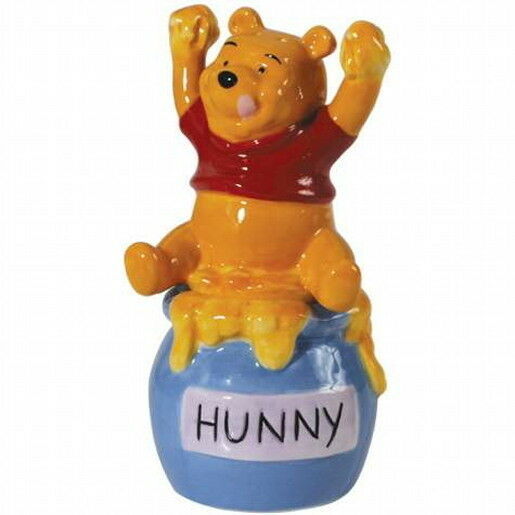This is an image of a shiny glazed ceramic figurine of Winnie the Pooh, with a completely white background. Winnie the Pooh, wearing his traditional red shirt that extends halfway up his stomach, is sitting on a light blue honeypot. The honeypot features a white banner with black capital letters spelling "H-U-N-N-Y." Honey is overflowing from the jar, spilling down its sides and in front of it. Winnie the Pooh's tongue is sticking out from the right side of his smiling face. Both of his legs are sticking straight out, and his arms are raised in the air, each holding globs of honey. His joyful expression is highlighted by his protruding tongue and playful posture.